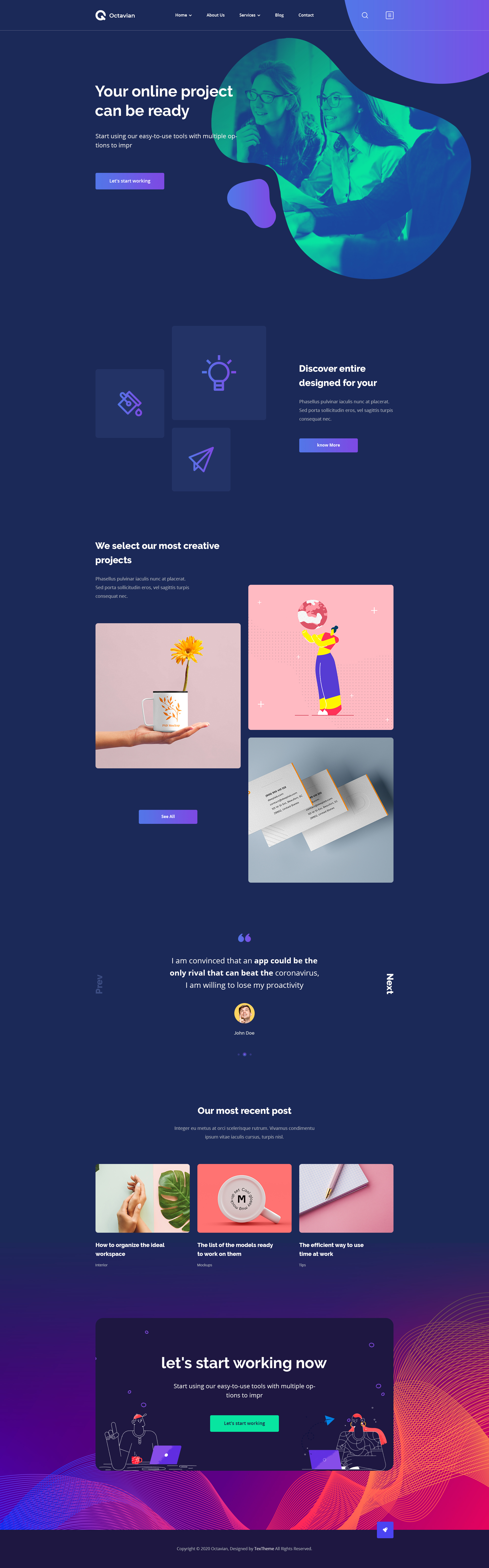The image is a vertically oriented rectangular box with a predominantly purple or dark blue background and small white text. At the top, there's a header containing a menu with words that are too small to decipher. Beneath this header, the phrase "Your online project can be ready" is clearly visible. Just below, a purple box with white text prominently stands out. 

In the middle of the image, a distinctive oblong, amoeba-shaped figure filled with people in a greenish hue catches the eye. Additionally, a purple quarter circle enters the frame from the top right corner. 

Approximately a third of the way down from the top, the image features three smaller boxes. Each box contains a different icon: a light bulb, an arrow, and a printer, respectively. To the right of these icons, there is some more small, unreadable text along with another purple box featuring small, indistinguishable writing inside.

Further down, three additional boxes are depicted, showing varied illustrations: a hand holding a cup with a flower emerging from it, a stack of envelopes, and what appears to be a clown holding a ball, although this last image is somewhat ambiguous.